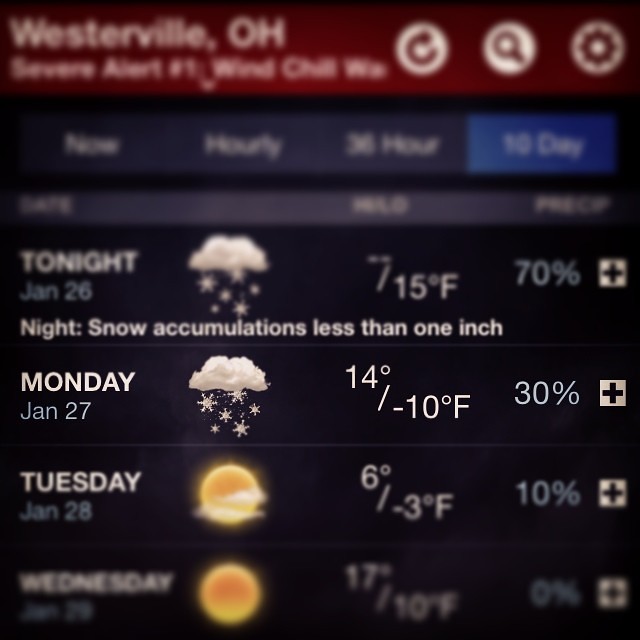The image is a color screenshot from a smartphone or tablet displaying a weather app in portrait orientation. At the top, a red strip stretches horizontally with white text reading "Westerville, Ohio." This strip includes a "severe alert" and "windchill" notification, along with navigation symbols: a back arrow, a magnifying glass, and a gear icon in white. 

Below is a section with a gray background and options for viewing the weather forecast: "Now," "Hourly," "36 Hour," and "10 Day," with the "10 Day" option highlighted in blue. The forecast details are shown beneath this, starting with "Tonight," followed by dates from Monday, January 27th to Wednesday, January 29th. Each date includes weather icons—clouds with snowflakes for most days and sun with clouds for Tuesday and Wednesday—along with temperature forecasts and precipitation percentages. Notably, Monday, January 27th, shows a cloud with snow, temperatures of 14°F and -10°F, and a 30% chance of precipitation. The overall screenshot is somewhat blurry but provides clear critical weather details.